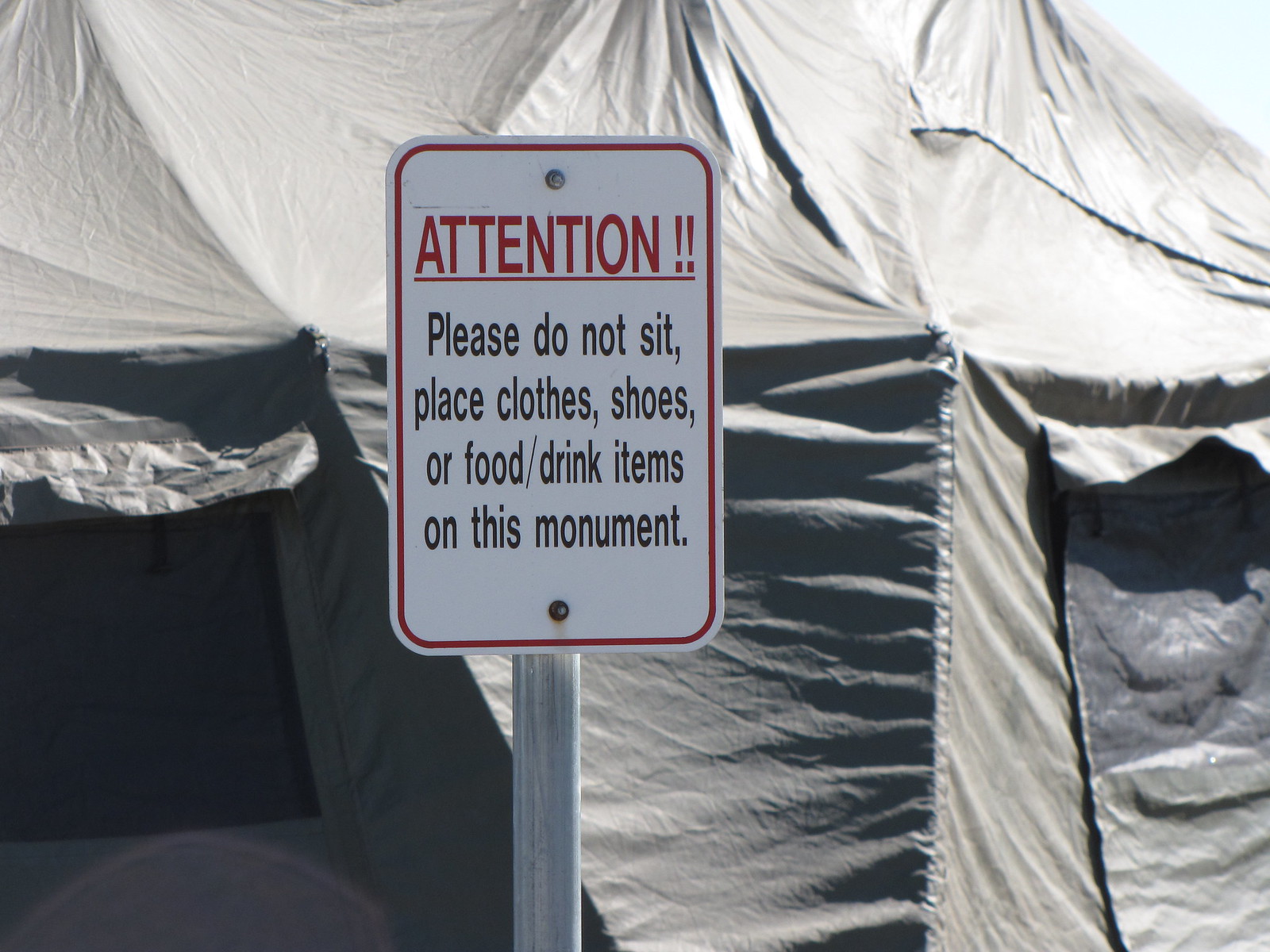In this image, a tall, vertical street sign is prominently displayed, anchored by two large steel bolts to a gray metal pole. The sign, with a white background framed by a red border, bears the bold red capitalized word "ATTENTION!!" followed by an important instruction in black text: "Please do not sit, place clothes, shoes, or food/drink items on this monument." The surrounding area reveals a setup of large canopies or tents, some with window-like openings and flaps made of either taut canvas or possibly nylon material. These tents, tinted in shades of olive and tan, cover a monument, which isn't fully visible due to the coverings. The sun casts light in the scene, illuminating the setup with blue skies in the background. The tents, marked by their ridges and wrinkles, suggest a structured yet temporary shelter over the enigmatic monument, seemingly indicating it is not a place for casual use.